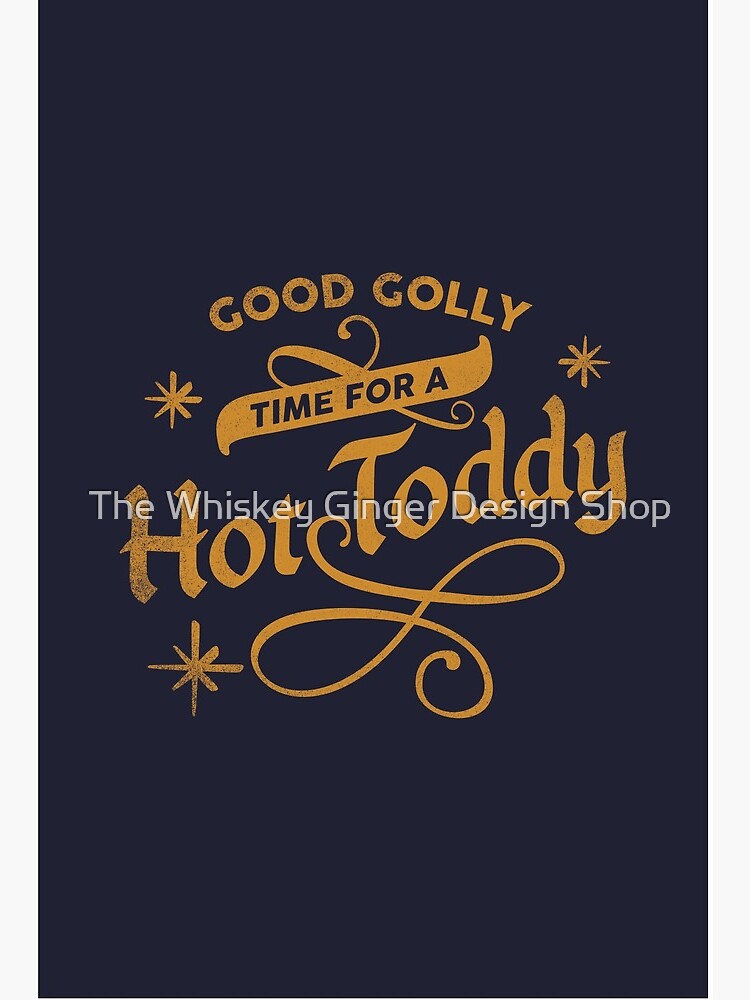This image is a digitally designed sample invitation cover from the Whiskey Ginger Design Shop. The design features a dark navy blue or black background with gold-yellow lettering and embellishments. The main text, "Good Golly, Time for a Hot Toddy," is stylishly arranged with "Good Golly" at the top in a slight arch. Below it, a slightly tilted gold banner hosts the words "Time for a," and "Hot Toddy" is prominently displayed in a larger, script-like font beneath the banner.

The design includes decorative elements like golden eight-pointed stars placed around the text, with three notable stars positioned above and below the words, adding to the festive feel. Additionally, elegant gold flourishes accentuate the banner and the phrase "Hot Toddy," with a scroll-like embellishment creating a visual connection between the words.

Overlaying this design is a white watermark reading "The Whiskey Ginger Design Shop," ensuring the sample image cannot be copied or stolen. The overall layout suggests it could be used as a phone background or a sophisticated printed invitation, with a touch of distressing on the gold lettering and stars to add a vintage aesthetic.